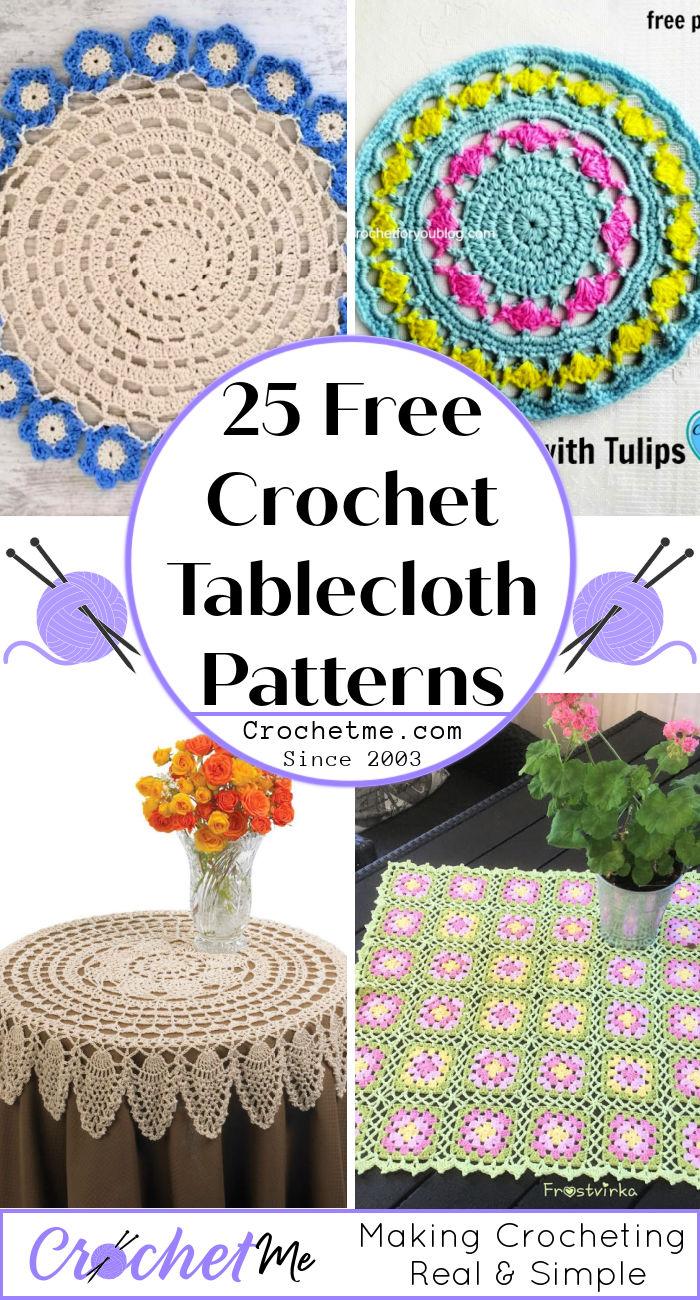This image features a portrait-oriented advertisement for a crochet website, CrochetMe.com, established in 2003. The centerpiece is a white circle with a purple border that prominently reads in black text, "25 Free Crochet Tablecloth Patterns," with a subheading, "CrochetMe.com since 2003," and the slogan "Making Crocheting Real and Simple" at the bottom.

Surrounding the circle, there are four detailed photographs showcasing different crochet designs. Starting from the top left, there is a cream-colored crochet with blue floral trim. To the top right, there's a vivid aqua crochet adorned with rings of yellow and pink, labeled "Tulips." In the bottom left, a table is elegantly set with a cream-colored crochet tablecloth, accentuated by a vase of orange flowers. In the bottom right, a lime green crochet featuring repeating square patterns in pink, purple, and white, is topped with a flower pot flaunting green leaves and pink flowers.

The overall visual style combines photographic realism with clean, modern graphic design elements, making it an attractive advertisement likely intended for a website, book, or magazine.